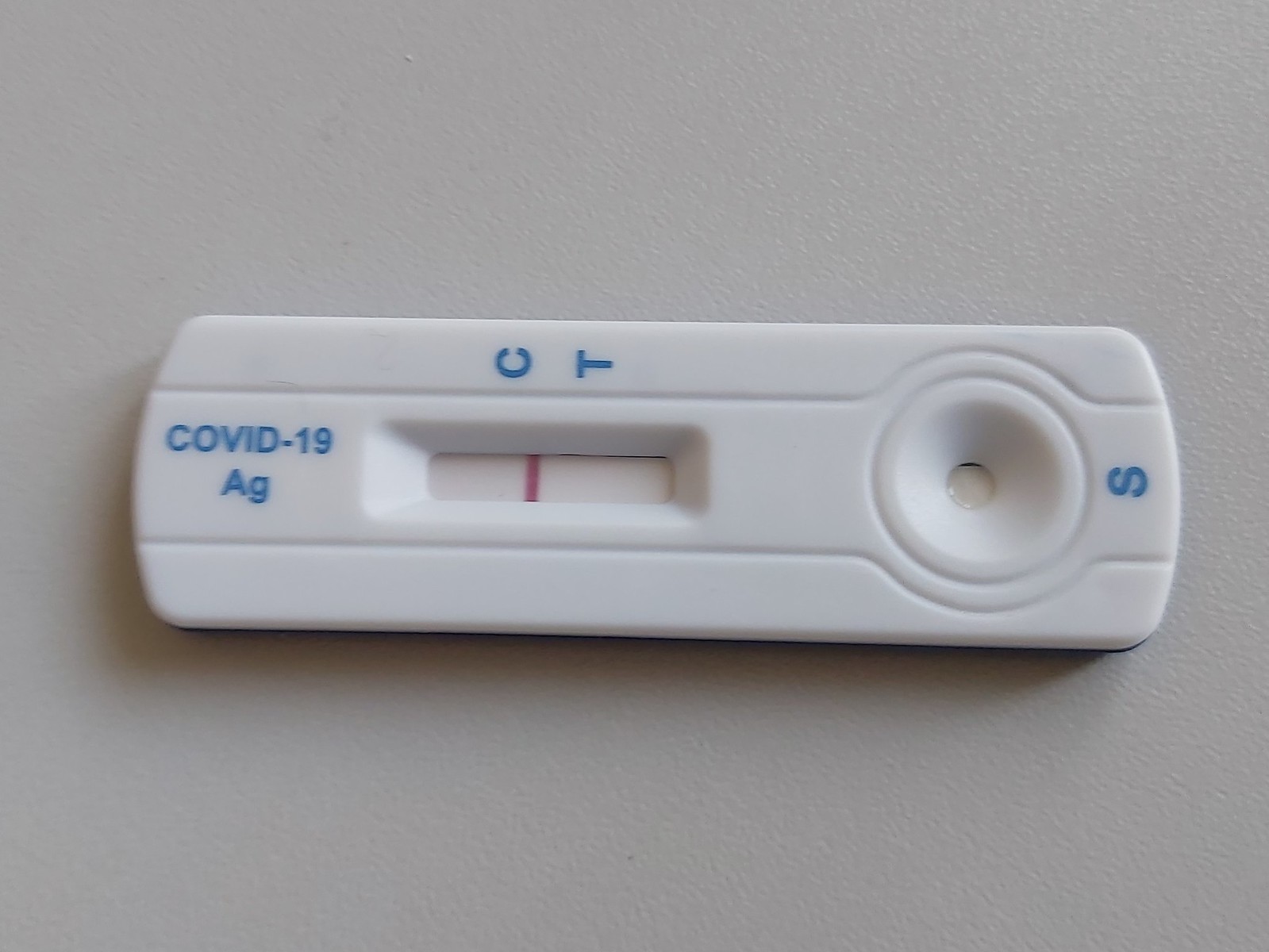In this photograph, we see a COVID-19 antigen testing device prominently placed on a solid white surface. The test kit is composed of a durable hard plastic, ensuring its sturdiness. 

On the left-hand side of the device, the label "COVID-19 AG" is clearly visible. Moving to the right, there's a small rectangular viewing window with a white background where test results are displayed. This window shows a single red line next to the letter "C," indicating a negative result for COVID-19. If the person were positive for COVID-19, two red lines—one next to "C" and the other next to "T"—would appear in this window.

Further to the right, there is a small circular collection spot, marked with "S," where a specimen is deposited. The process for using this kit involves swabbing the mouth, placing the swab in a reagent container, and then adding the liquid to the collection spot on the test strip.

This particular test kit is of medium size, larger than many standard kits, making it easy to handle. It serves as a typical COVID-19 testing kit, used to determine if a person is infected with the virus. The image is clean and focused, showcasing the essential components needed to understand the use and function of the testing device.